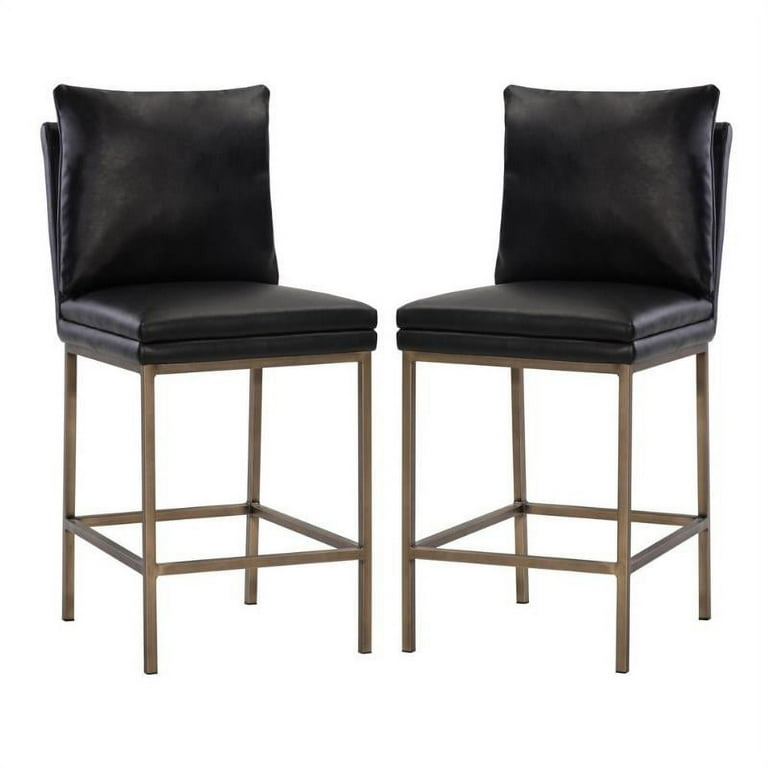The image depicts two elegantly designed high-end chairs, both positioned centrally and slightly facing each other. These chairs stand on a sleek, coppery or bronze-colored thin metal frame, which includes four straight legs with no ornate designs. A square base at the bottom acts as a footrest. The chairs feature double-layered black leather cushions for added comfort, with one cushion for the seating area and another for the backrest, ensuring ample support. The backrest is further enhanced with two black throw pillows. The overall setting and style of the image emphasize the chairs as sophisticated furniture products, all set against a clean, white background.